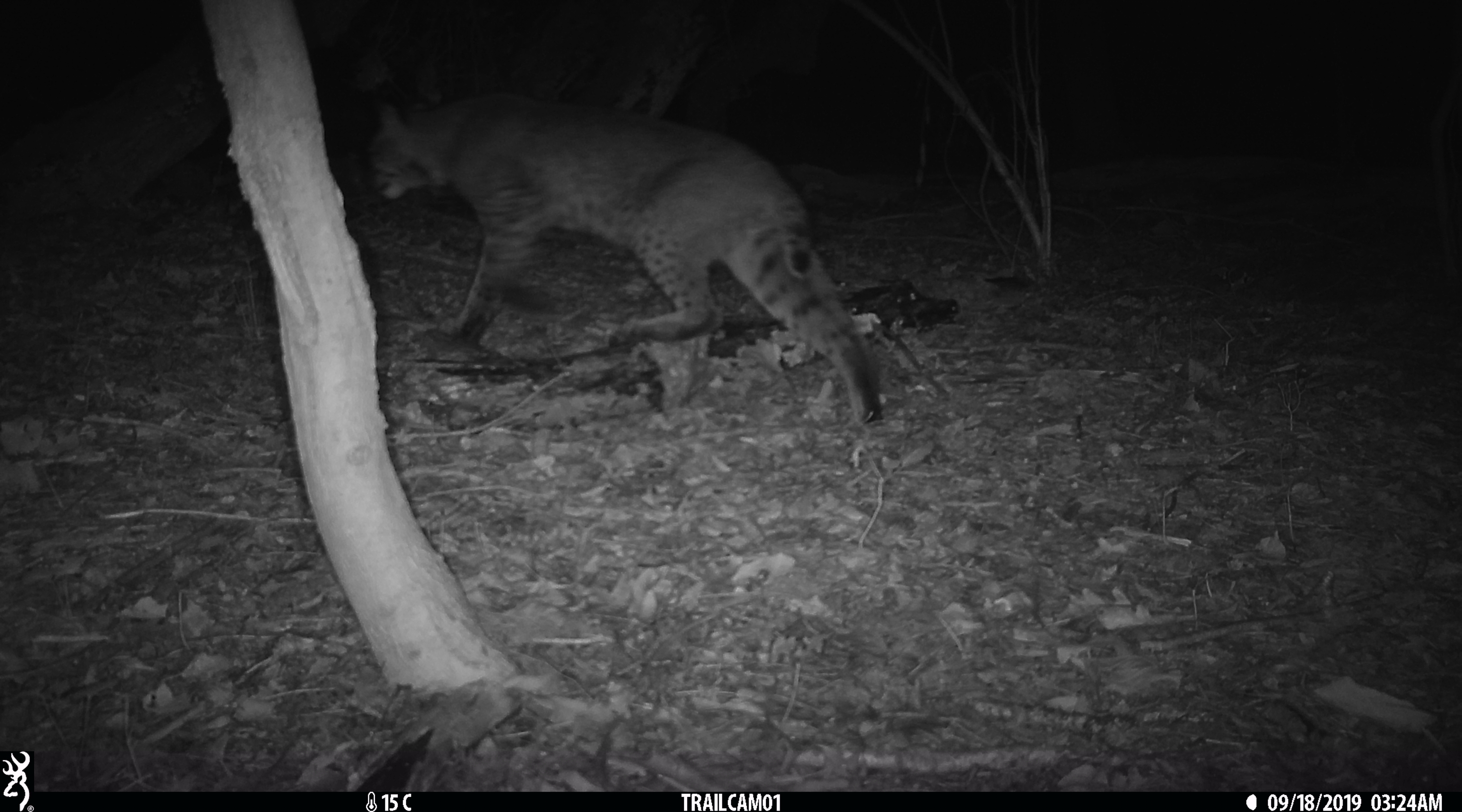In this black-and-white still captured by a trail camera at night in the woods, the ground is densely covered with leaves and sticks. The image reveals a stark, leafless tree on the left side, its branches reaching upward and slightly leaning left. Near the top center of the frame, a jaguar is spotted walking away from the camera. Its head is turned to the left and slightly back, with its rear end more prominently visible to the right and closer to the camera. The jaguar’s front leg is on the ground, while its left back leg is lifted as if in mid-stride, and its right leg is pushing off the ground. The jaguar’s short tail and distinctive brown fur with black stripes are evident. 

The bottom of the photograph features a thin black bar with "15C" in white lettering just below the 'T' on the left side, indicating the temperature. In the center of this bar is the label "TRAILCAM01," identifying the type of camera used. On the bottom right corner, the timestamp shows the date "09-18-2019" and the time "3:24 AM," marking the moment this nocturnal scene was captured. The overall atmosphere is dark and mysterious, emphasized by the nighttime setting and the partially obscured view of the jaguar, which adds to the intrigue of this woodland encounter.